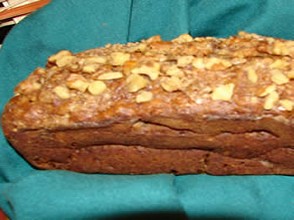The image features a rectangular-shaped loaf of bread, sitting on a teal or greenish-colored cloth that could be parchment or fabric. The bread itself is golden brown, with a slightly flat top and noticeable indentations and grooves on the sides, suggesting it was folded over itself during preparation. The top of the loaf is adorned with what appears to be an assortment of light-colored nuts or possibly pieces of fruit, which are irregularly shaped but predominantly square or round. These toppings are scattered generously, though they do not fully obscure the bread's surface. Positioned in what seems to be a kitchen setting, you can discern a wooden-edged counter or table in the top left of the image. The potential white wall and some black elements in the background provide subtle context of a homey, rustic environment. The bread looks freshly baked and invites the viewer to imagine enjoying a slice.